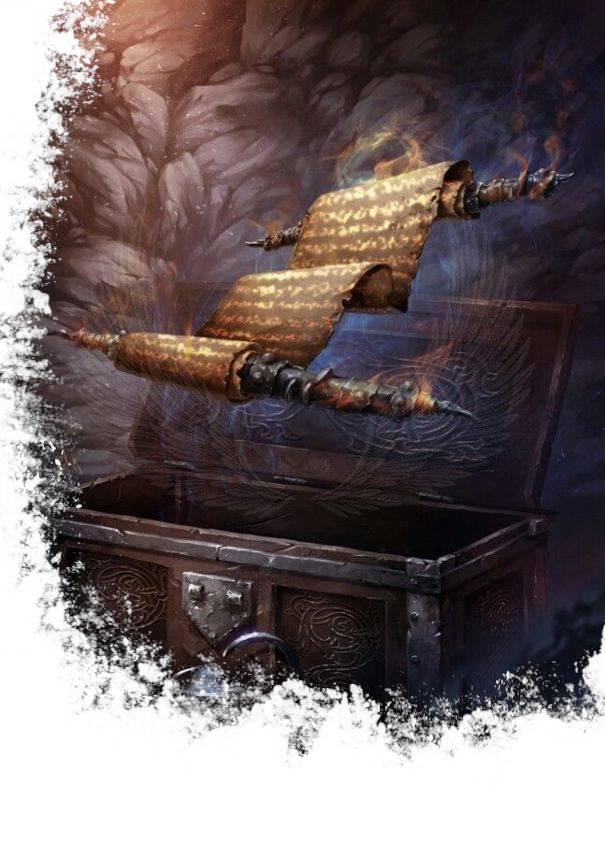This digitally illustrated, color artwork presents a mystical scene with a unique, non-rectangular frame. The top and right sides of the image are defined by straight lines, while the left and bottom edges appear to be fading away, as if partially erased or gradually blending into the canvas. This gives the artwork a dynamic and ethereal aesthetic, resembling an image that's either materializing or dissolving.

At the center of this fantasy illustration, a dark brown treasure chest with ornate embossing, metal detailing, clasps, and rivets sits open. The chest, with its gothic appearance, has its lid tilted back, revealing a floating, loosely unfurled scroll. This scroll extends diagonally to the right, with portions still wrapped around its rollers. The parchment looks aged and weathered, adorned with shimmering golden runes that hint at an indecipherable, possibly invented language.

The background features swirling bands of silvery and grey smoke, enveloping the entire scene and enhancing its otherworldly atmosphere. The overall style of the artwork is highly stylized, reminiscent of video game or comic book art, with an emphasis on the ancient and arcane.